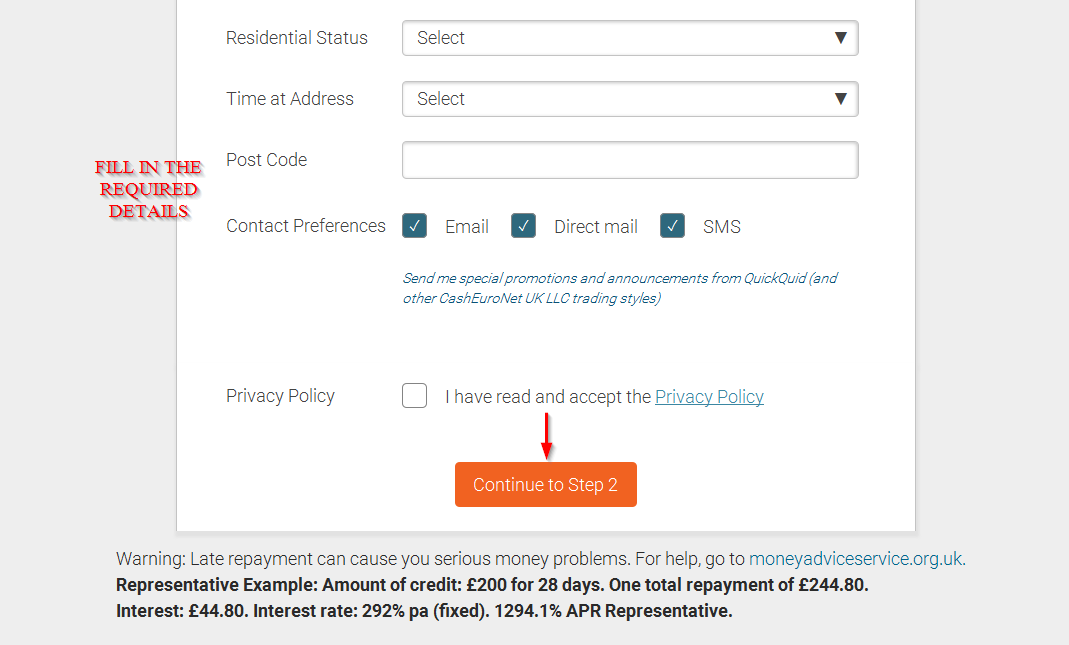The image depicts a form on a website or app with a gray background. On the left side, there is red text that reads "Fill in the required details." Adjacent to this is a white box labeled "Residential Status" featuring a drop-down menu with the default option "Select." Below that, another drop-down menu labeled "Time at Address" also shows "Select" as the default choice. Following these, there is an empty input field for a "Postcode." 

Under the contact preferences section, options for "Email," "Direct Mail," and "SMS" are available, each accompanied by checkboxes that are already checked. A promotional message underneath reads, "Send me special promotions and announcements from QuickAid and other CashEuronet UK LLC trading styles." 

Further down, a checkbox next to the text, "I have read and accept the privacy policy," is also provided. Beneath this, a red arrow points downwards towards a button that says "Continue to Step Two." 

At the bottom of the form, there is a warning stating, "Warning: Late repayment can cause serious money problems. For help, go to moneyadviceservice.org.uk." A representative example follows: "Amount of credit: £200 for 28 days. Total repayment: £244.80 (Interest: £44.80). Interest rate: 292% PA fixed or 1294.1% APR representative."